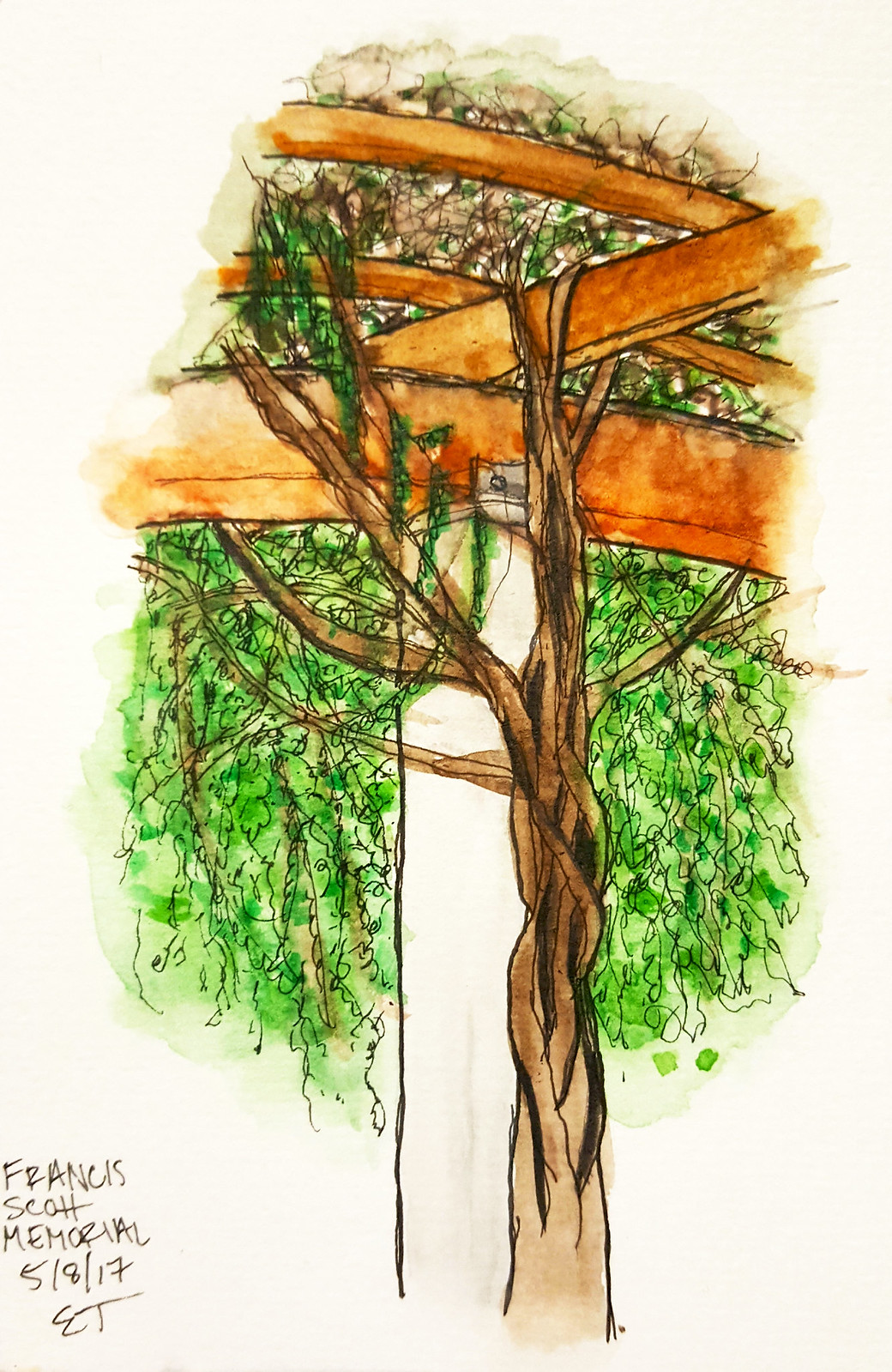This is a detailed artist's drawing on very light, white-colored paper, depicting a tree that has grown around a pole. The pole is affixed to four large wooden beams – three oriented horizontally from left to right, and one positioned at a slight angle. The setting appears to be an outdoor area, suggesting it might be part of a porch structure.

The tree's trunk is solid at the base but branches out as it ascends, with the thicker branches intertwining around the wooden beams rather than through them. The thinner branches are depicted with squiggly lines and are adorned with light green leaves. The background at the top of the drawing has a hint of gray shading.

In the bottom left corner, there is a handwritten note that reads "Francis Scott Memorial 5/8/17," followed by the capital letters "E.T."